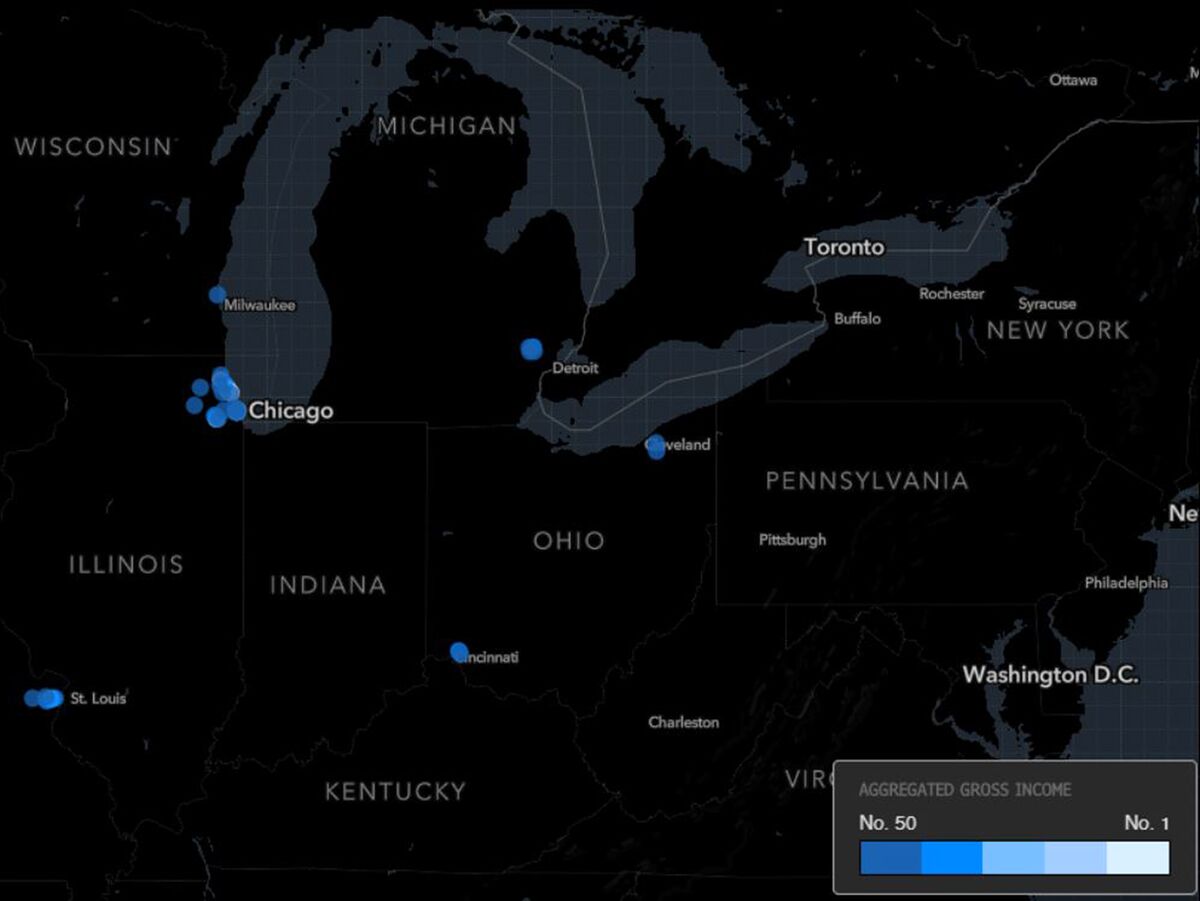The image appears to be an interactive map or diagram depicting the United States and Canada in stark black silhouettes, with significant bodies of water, including the Great Lakes, rendered in light grey. The map is dotted with colored bubbles, predominantly focused around Chicago, but also scattered across cities like St. Louis, Cincinnati, Detroit, Cleveland, and Milwaukee. These bubbles vary in shades of blue, ranging from nearly white (which represents rank number 1) to dark blue (which signifies rank number 50), according to a legend located in the bottom right-hand corner of the map. This legend indicates that the colors correspond to levels of aggregated gross income, though the specific nature of this income and the entities or individuals represented by the bubbles remain unidentified. The distribution and overlay of the bubbles make exact interpretation challenging, particularly due to the zoom level of the map.